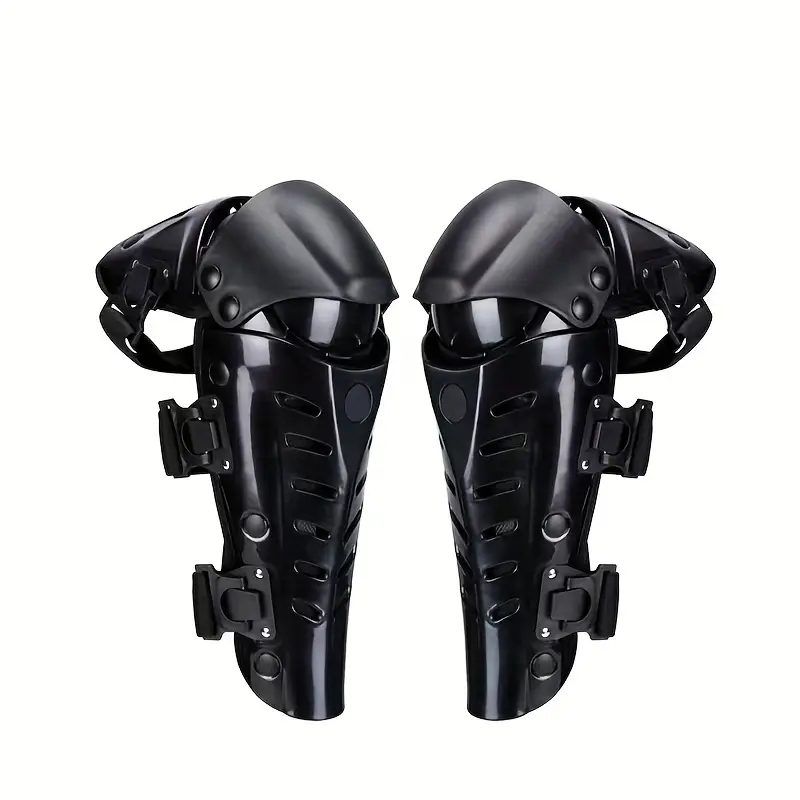Set against a plain white background, the image showcases two black leg guards designed for heavy-duty protection, likely for activities such as motorcycling or sports. The leg guards are symmetrically positioned, with the one on the left turned slightly to the right and the one on the right angled slightly to the left, giving the impression that they are facing each other. Each guard consists of three main components: a thigh protector running parallel along the upper leg, a knee cap section featuring an additional casing for enhanced protection, and a shin guard extending down to the ankle. The guards are equipped with three adjustable straps for securing them in place and feature a series of six horizontal slits on the shin area for ventilation. The hard, black plastic shell offers robust protection, and the interconnected pieces allow flexibility while maintaining structural integrity through a bolted system. The design is both functional and aesthetically futuristic, tailored to provide comprehensive leg coverage and breathability.